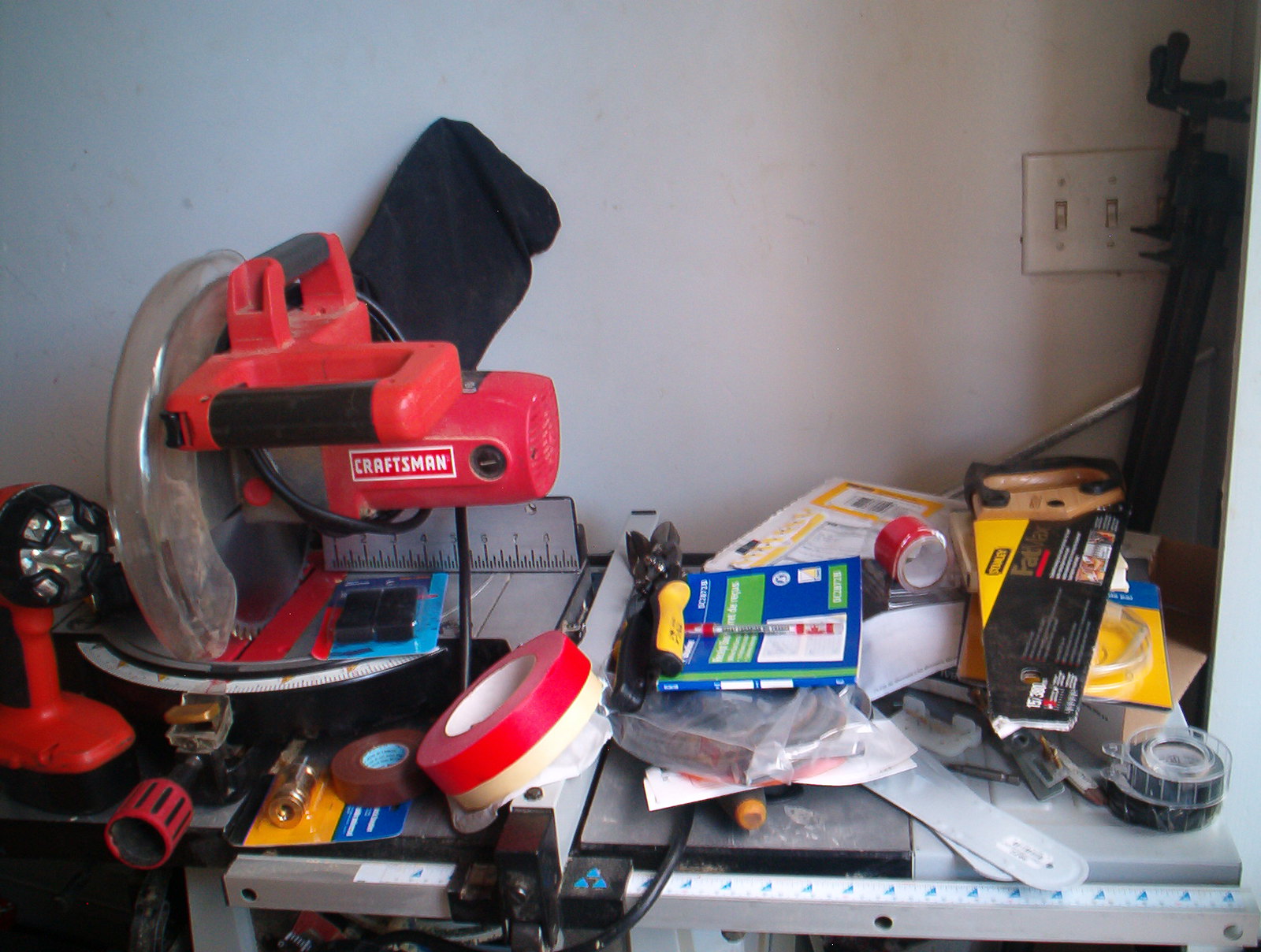This indoor photograph captures a well-lit workspace with illumination coming from a window on the right-hand side, evident from the bright light and visible window frame. In the top right corner, the image features two light switches mounted on a backing panel, alongside an indeterminate object leaning against the wall. The walls, painted white, acquire a slight peach hue in the direct light and transition to a greyish shade in the shadows. The bottom half of the photograph is dominated by a robust workbench constructed from a metal frame, laden with various tools and materials. Prominently featured on the workbench is a red circular saw table equipped with a dust collection bag. To the bottom left, a red power drill or similar tool is visible. The cluttered surface of the workbench is scattered with an assortment of items including different types of tape, packaging with brass components, potential sandpaper, various papers, and metal rulers, showcasing a busy and functional workspace.